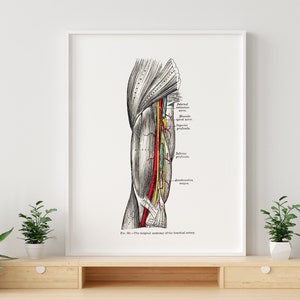The image depicts a home decor setup featuring a light beech wood table with a small shelf that has two drawers adorned with white knobs. Centrally positioned on the table is a framed picture, resembling a page from an anatomy book—possibly Gray’s Anatomy—displaying an anatomical diagram of the upper arm, from just below the shoulder to above the elbow. The diagram is detailed, with the major artery, likely the brachial artery, highlighted in red, and includes yellow accents that may indicate nerves. This anatomical rendering is in shades of black and white with white highlights, all set against a white background within a white frame. Flanking the framed picture are two green house plants, possibly ficus or ferns, each in white vases. The overall setting is indoors, with the scene backed by a white wall. The colors in the image include hues of white, yellow, brown, and green from the various elements.